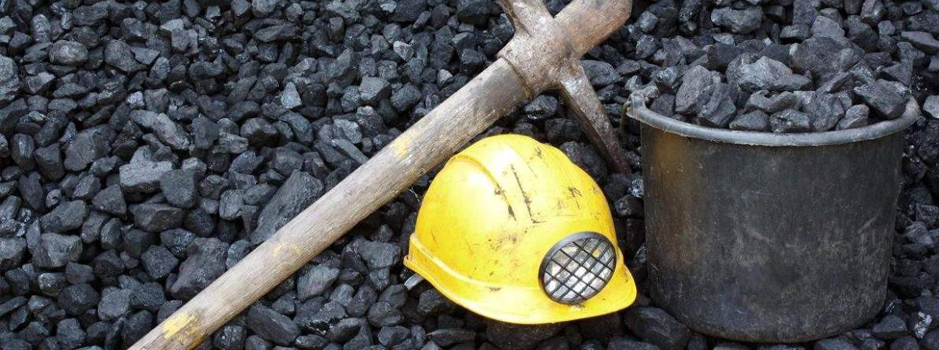The image showcases an evocative scene reminiscent of coal mining, artfully arranged to emphasize the theme. Dominating the frame is a substantial mound of coal that fills the entire image, contrasting starkly against the stone flooring beneath it. Central to the composition is an older metal bucket, brimming with coal chunks. To the left of the bucket lies a yellow hard hat, fitted with a front-mounted light typical of mining helmets. Adjacent to this helmet, an antiquated wooden pickaxe rests against the coal, its metal head showing signs of rust. The overall setting appears to be outdoors, possibly on a railway track, with a blend of colors including black, gray, silver, light brown, yellow, and tan. This carefully arranged scene recreates the essence of a coal mining site using a limited yet impactful selection of mining tools and materials.